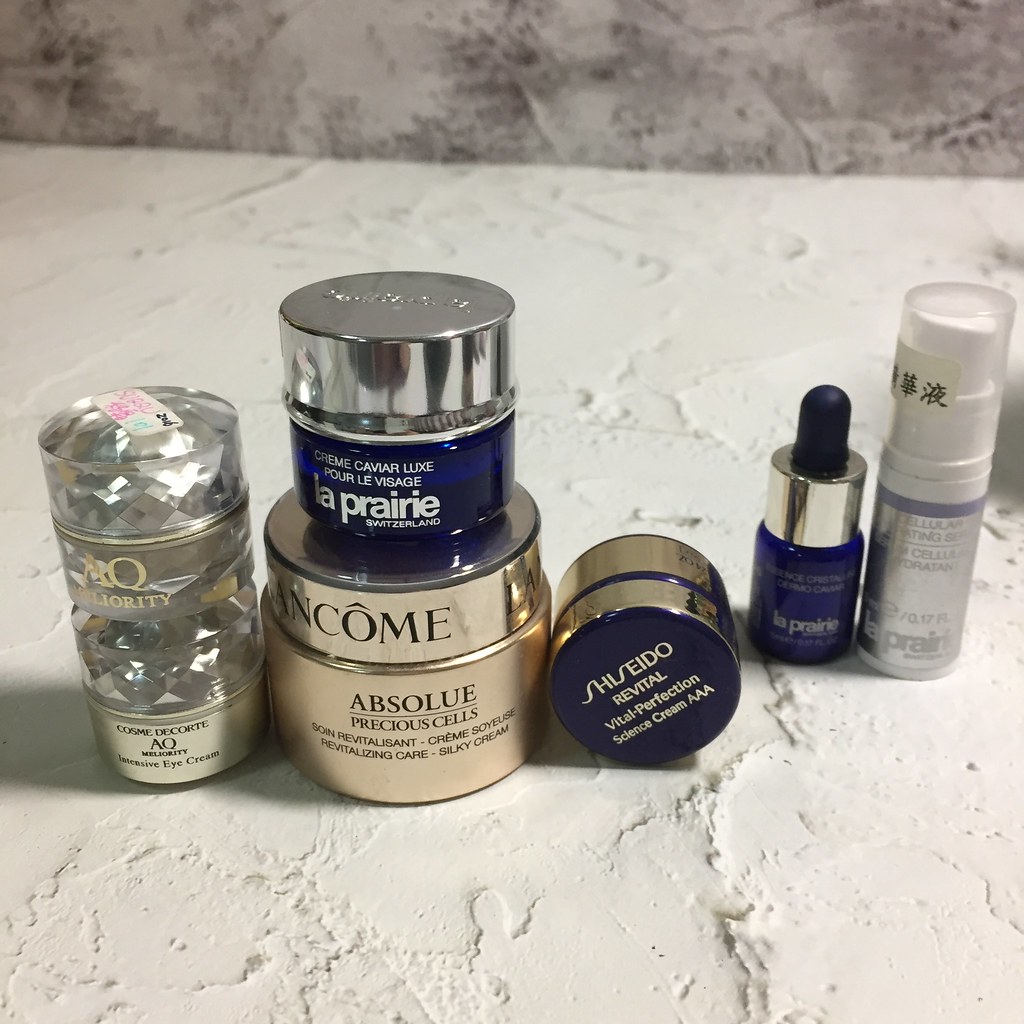This color photograph showcases an array of luxurious beauty supply items meticulously arranged on a thickly textured white surface, set against a background of a gray wall with some black areas. From left to right, the collection includes:

1. A sophisticated jar with a faceted silver lid labeled "AQ MELORITY COSME DECORTE Intensive Eye Cream."
2. A stylish jar featuring a gold color with a matching gold lid. The lid is inscribed with "LANCOME" in black lettering, while the front reads "ABSOLUE Precious Cells Revitalizing Care Silky Cream," with the French translation above the English.
3. Perched on top of the Lancome product is a compact blue jar with a silver lid, marked with "Crème Caviar Luxe Pour Le Visage LA PRAIRIE Switzerland" in white lettering.
4. An elegant, small, golden-colored pot lying on its side, with a dark blue lid inscribed with "SHISEIDO REVITAL Vital Perfection Science Cream AA."
5. A slender blue bottle capped with silver and featuring a black stopper. The partially visible label includes "LA PRAIRIE" at the bottom in white lettering.
6. A petite white bottle with a clear plastic cap, adorned with foreign Asian script alongside some barely legible English text. The bottom of the bottle prominently displays the name "LA PRAIRIE."

Each item not only represents some of the finest names in luxury skincare but collectively offers a lavish visual appeal against the minimalist and textured backdrop.